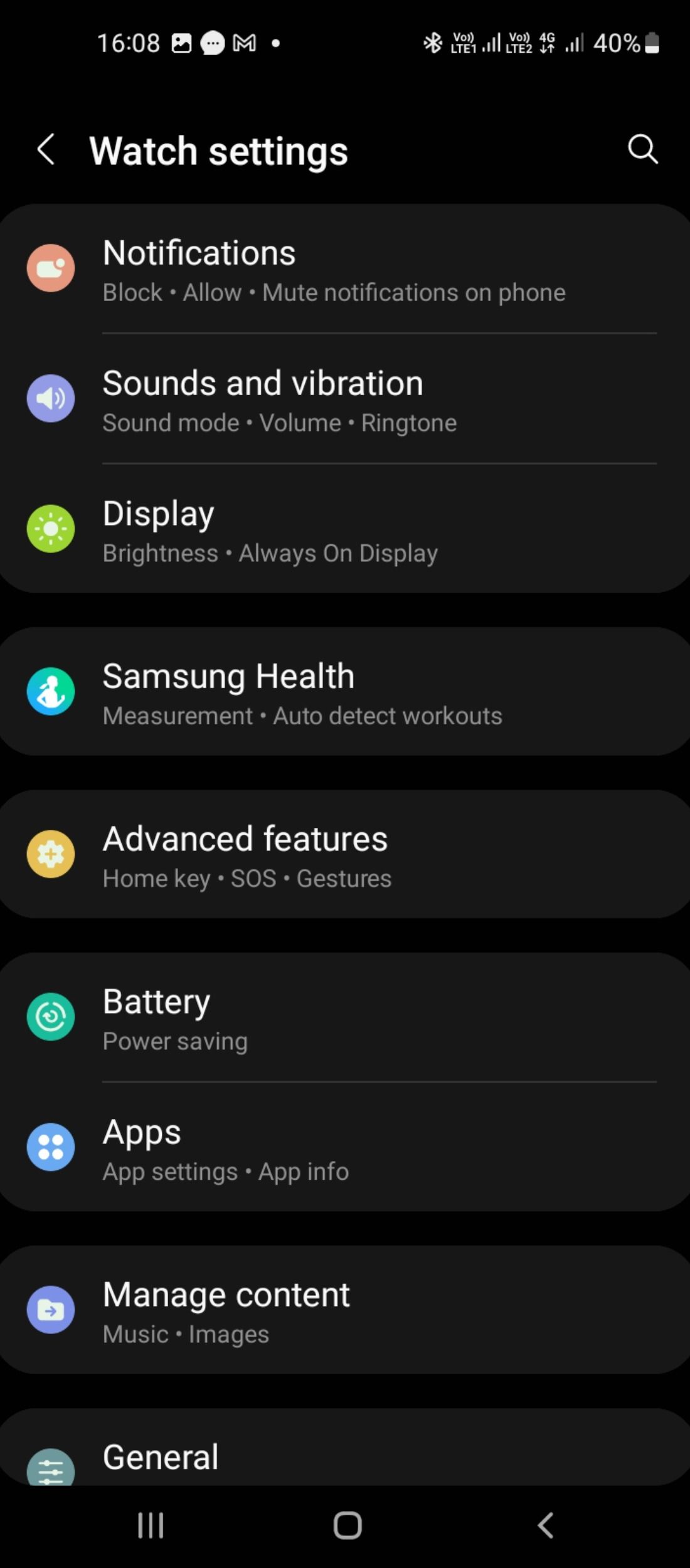This image features a screenshot taken from a smartphone, displaying the user’s watch settings interface, set against a black-and-white background. At the top, "Watch settings" is prominently displayed, accompanied by a search bar to its right. 

Below, a detailed list of settings is presented:
1. **Notifications**: Marked with an orange notification icon, offering options to block, allow, or mute notifications on the phone.
2. **Sounds and Vibration**: Identified by a purple sound icon, with sub-options for sound mode, volume, and ringtone management.
3. **Display**: Featuring a green circle icon with a sun, which includes settings for brightness and always-on display.
4. **Samsung Health**: Recognized by an icon of a running person, allowing auto-detection of workouts.
5. **Advanced Features**: Denoted by a yellow icon with a white flower, includes settings for the home key, SOS functionality, and gestures.
6. **Battery**: Highlighted with a green circular icon and arrows, offering power-saving options.
7. **Apps**: Containing sub-sections of app settings and app info, represented by a periwinkle-colored circle with four white circles inside.
8. **Manage Account**: Shown with a purple circle and a folder icon, linked to music and images.
9. **General**: This section features a gray circular icon but is partially cut off in the image.

Additional information visible in the screenshot includes the time, which reads 16:08, along with the 4G network signal and a battery level of 40%.